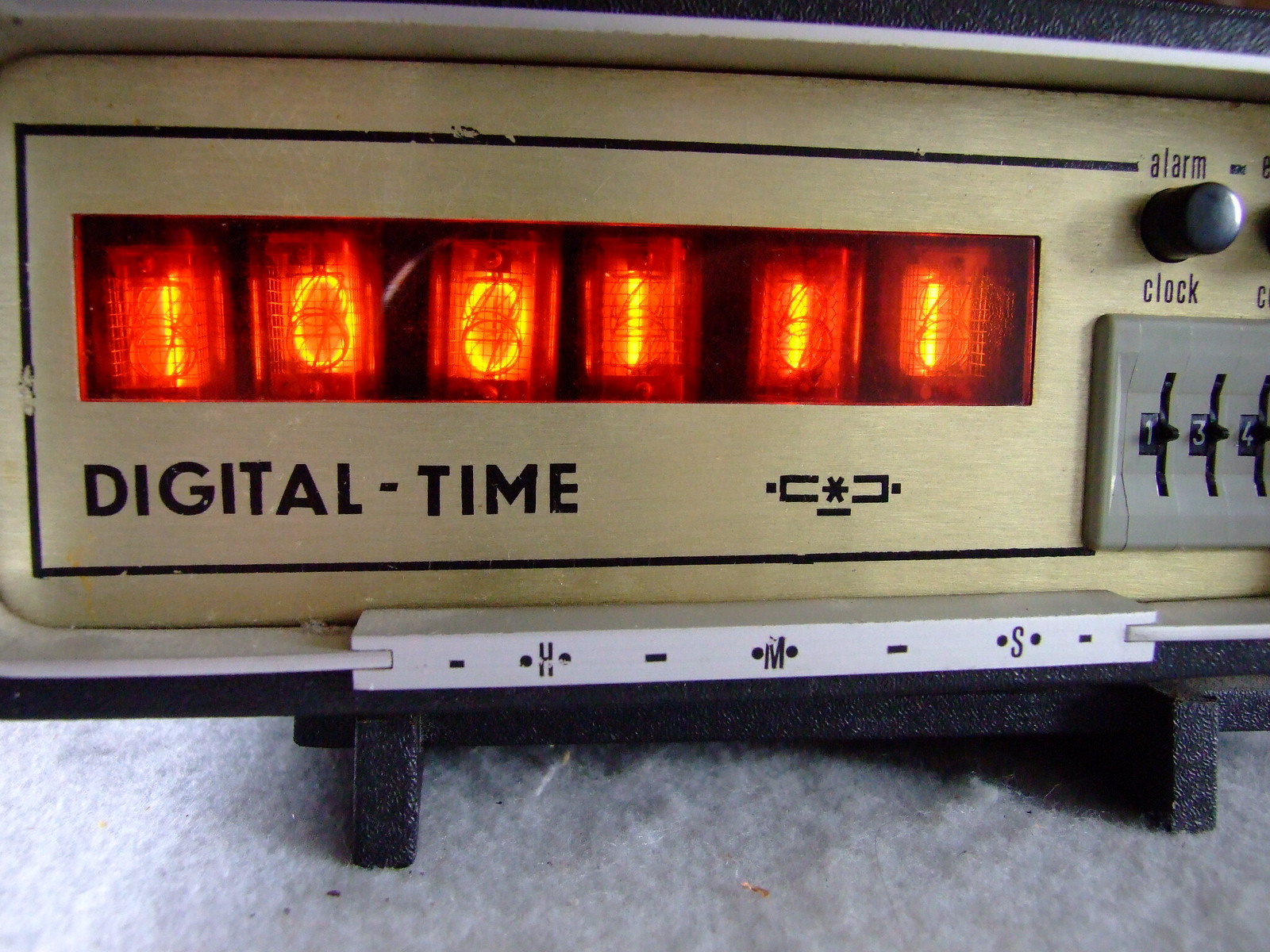A close-up photograph features an intriguing, old-fashioned alarm clock with a whimsical design reminiscent of a toaster. The clock is coated in a yellow-gold hue, which gives it a vintage appeal. Its digital display, illuminated with red light, shows the numbers "10:01:11," indicating the time as 10:01 and 11 seconds. Despite the digital display, the time is separated by a hyphen rather than the usual colon, a quirky detail that adds to the clock's retro aesthetic. 

On the right side of the alarm clock, there are several control buttons labeled "Alarm" and "Clock," allowing the user to set and manage the alert times. Below these controls are small, toaster-like slots, designed for numerals to be arranged manually, further emphasizing the clock's nostalgic charm. This hybrid of digital and mechanical elements evokes a sense of novelty, blending old-school construction with digital technology in a unique and detailed manner.